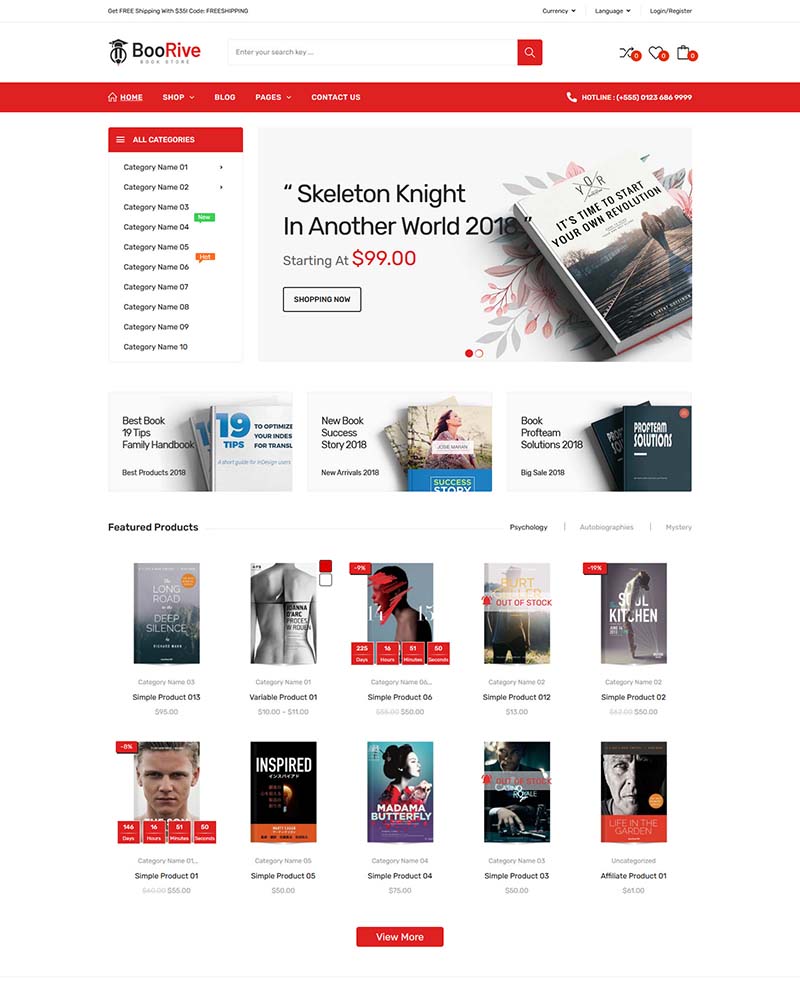**Detailed Descriptive Caption:**

The website features a clean, white background with an offer banner prominently displayed at the top of the screen that mentions "Get Free Shipping." On the far right, there are three additional categories, though their labels are not entirely visible. The first and second categories feature drop-down arrows for more options, with the second category seemingly labeled "Language." 

The header showcases the company name "Boorive," with "B-O-O" in black and "R-I-V-E" in red. Adjacent to the name is a circular logo resembling a globe with a graduation cap perched on top. To the right of the logo is a white search bar, followed by a red box containing a white magnifying glass icon. Further to the right are three icons: crisscrossing arrows within a red circle, a heart within a red circle, and a shopping bag within a red circle. 

Beneath the header, a red box with white text labeled "All Categories" leads into a list of categories in black text within white boxes. These include Category Names one through ten. 

To the right of the category list is an image promoting a product with black text that reads, "Skeleton Knight in Another World 2018." An introductory price of $99 is highlighted in red, alongside a call to action, "Shop Now." Accompanying this text is an image of a book titled, "It's Time to Start Your Own Revolution."

Next, a section with a white background adorned with gray and red flowers transitions into various book categories. Featured sections include "Best Book: 19 Tips Family Handbook," "New Book Success Story 2018" with an image of a book featuring a female, and "Book Protein Solutions 2018" showcasing a black book.

Below these sections, "Featured Products" is highlighted in black text. To the right, there is a segment labeled "Psychology," alongside two gray sections that are difficult to read. Featured products consist of ten books arranged in two rows of five. 

The first row of books includes:
1. A book with a long title.
2. A book depicting the back of a female.
3. A book featuring a black female with a red face.
4. A book showing a man in a suit.
5. A book in black and white that portrays a woman in a tiled soul kitchen.

The second row of books includes:
1. A book with a clean-shaven Caucasian male staring directly at the viewer.
2. A book titled "Inspire" with a black cover.
3. "Madame Butterfly," featuring a geisha lady in a red coat, traditional hairstyle, and white makeup.
4. "Casino Royale," displaying the movie poster of Daniel Craig at a poker table with his gun.
5. A black and white book showing half of a male's face.

At the bottom, a red button with white text invites users to "View More."